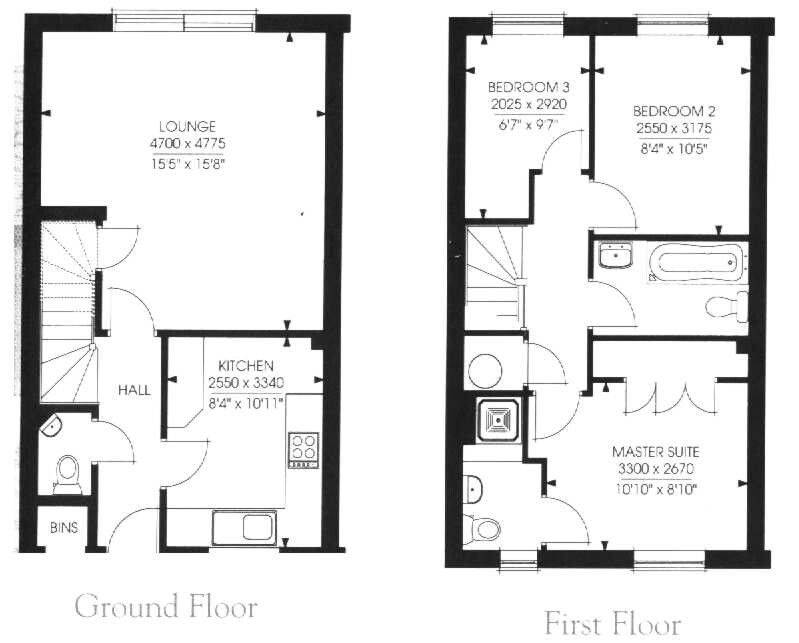This image showcases a detailed blueprint of a home layout, divided into two distinct sections: the ground floor on the left and the first floor on the right, each clearly labeled at the bottom of the diagram. 

On the ground floor, the lounge room is prominently displayed, measuring 155 feet by 15 feet 8 inches. Adjacent to it, in the bottom right corner of this section, is the kitchen, precisely sized at 8 feet 4 inches by 10 feet 11 inches. The kitchen is well-equipped with essential appliances, including a stove and a sink. Various other areas are depicted with open and closed doors, illustrated through curved lines indicating their swing direction. Notably, there is a bathroom positioned to the left side of the layout, and bins are located at the very bottom-left corner. Additionally, near the bathroom in the hallway, a set of doors leads to stairs, presumably connecting the ground floor to either a basement or the first floor.

The first floor, presented on the right section of the image, comprises three bedrooms: Bedroom 2, Bedroom 3, and a master suite with its own bathroom strategically positioned in the middle. This comprehensive blueprint provides a clear and meticulous representation of the home's layout for easy visualization and understanding.